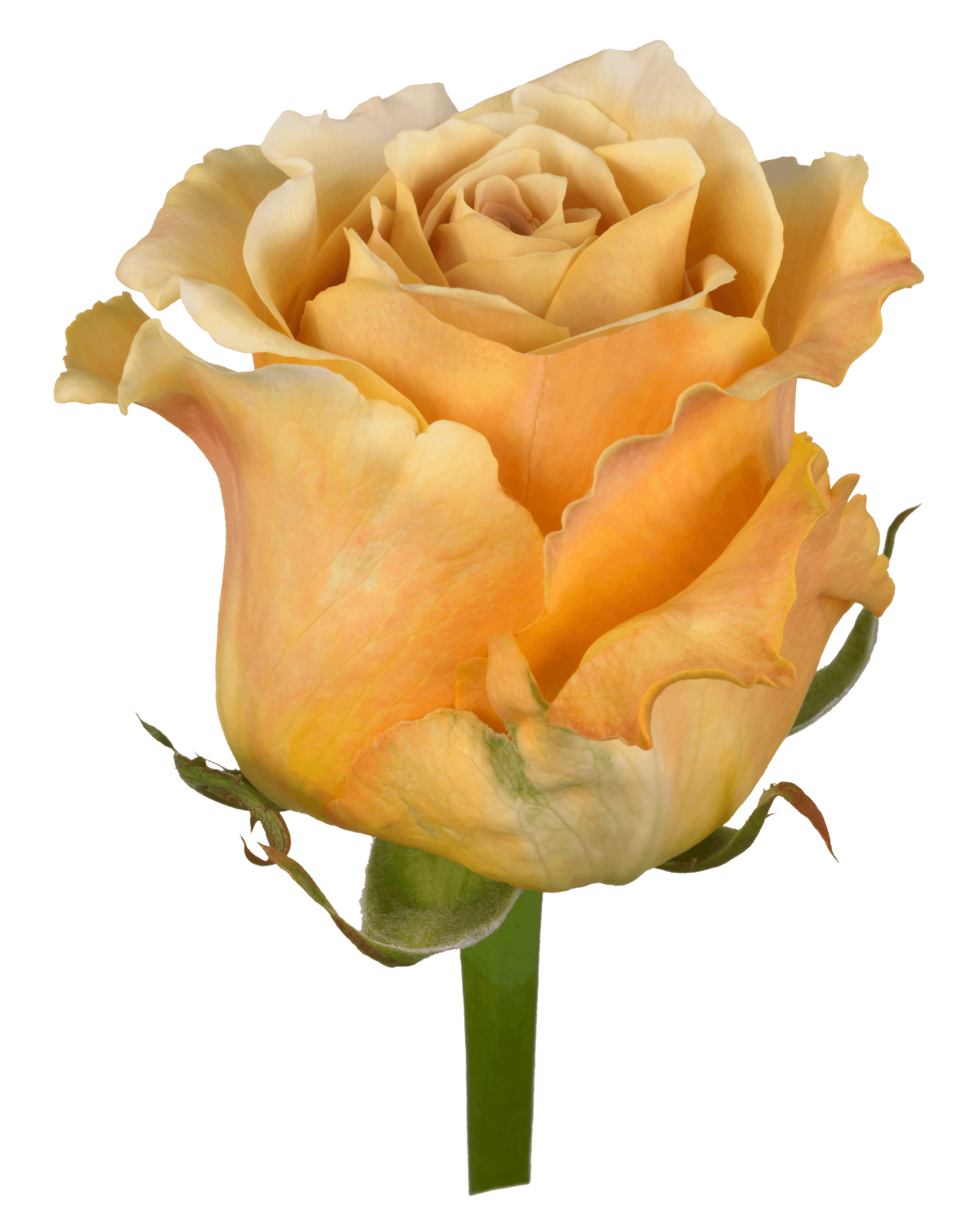This is a close-up photograph of a yellow rose, captured against an entirely white background. The rose itself is very full, with petals that are predominantly dark yellow, transitioning to a lighter yellow at the tips. Some petals have hints of light green near the base of the flower. The edges of the petals are slightly curled and look a bit wrinkly, characteristic of a freshly picked rose. The green stem is visible at the bottom of the image, along with a couple of curved blades that extend to the right and left. One of these blades features a touch of red at its end. The overall composition focuses solely on showcasing the elegance of the rose, with no text or other distractions present in the image.